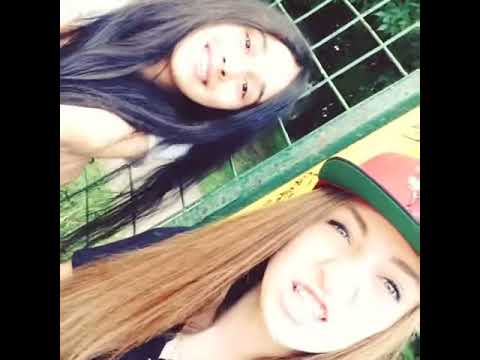The photograph depicts two young women, appearing to be around 13-14 years old, captured in a somewhat blurry, selfie-style image oriented at an angle. The image is framed by thick vertical black borders on both sides. To view it correctly, one needs to tilt their head to the left. The young woman positioned at the top left, who appears higher in the image, has long, straight black hair draped over her shoulders. She is smiling broadly, displaying her teeth. The second young woman, located in the lower right corner of the image, has long, straight strawberry blonde hair. She is wearing a red and green baseball cap and a dark-colored t-shirt that's partly obscured by her hair. Her mouth is open in what seems to be a displeased or disgusted smile, also showing her teeth. Behind them, a green-framed window with small panes and possibly a yellow pillar can be seen, but much of the background is obscured by their presence.